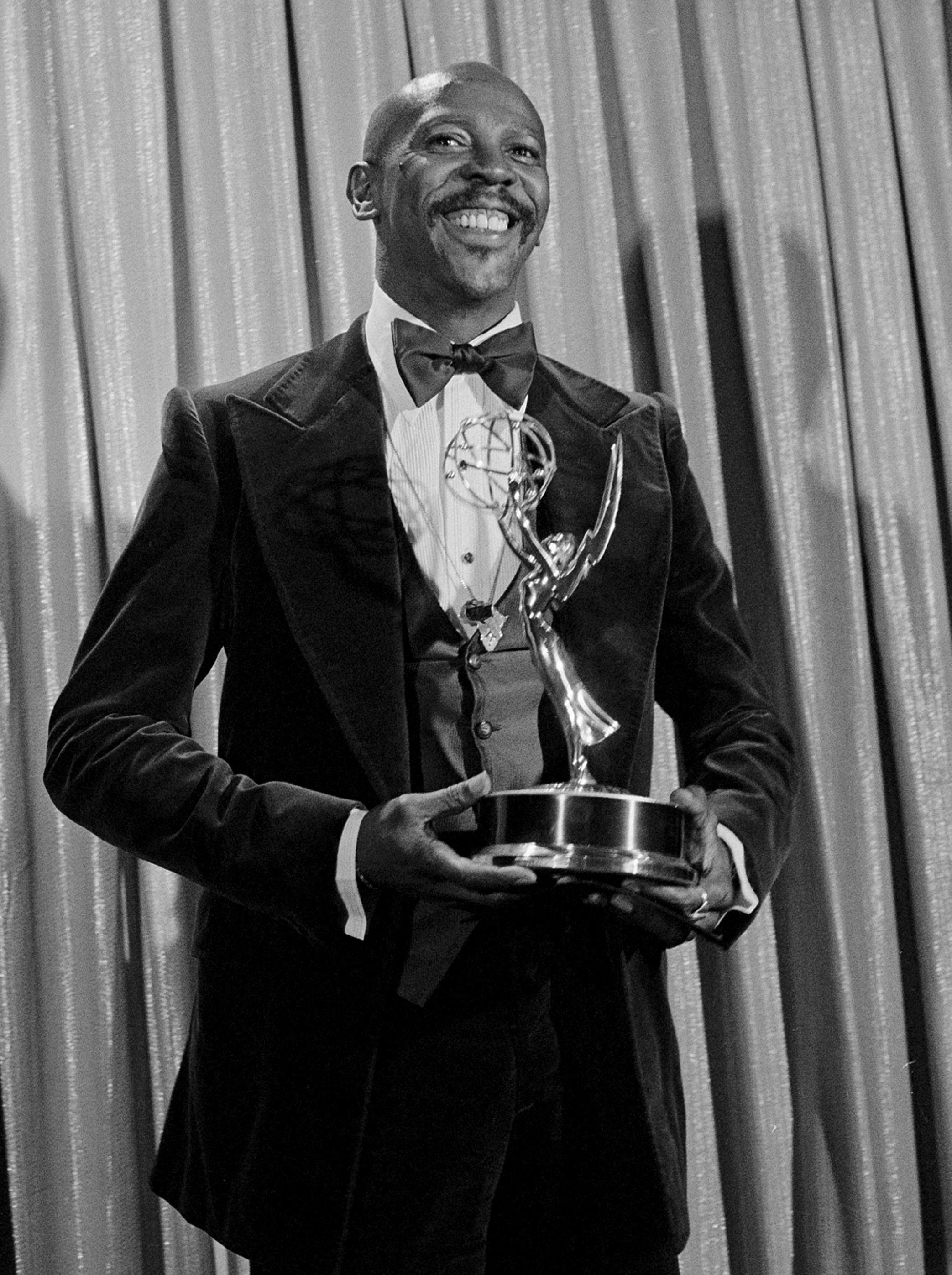This black-and-white photograph captures a young African-American male, likely in his early 30s, who strongly resembles a young Louis Gossett Jr. He has a shaved head and a mustache, and he is beaming with a wide smile as he holds an award in both hands at chest height. The award depicts a woman with wings, reaching up to hold a circular object, and appears to be gold or metallic. The setting suggests an entertainment awards program from the 1970s, potentially the Golden Globe Awards. The man is impeccably dressed in a 1970s-style black tuxedo that includes a large black bow tie, a traditional white shirt with black buttons, a black vest, and black pants. His white cuffs extend about half an inch from his jacket sleeves. He is also adorned with a chain necklace featuring a pendant and wears a ring on his left pointer finger. Behind him, a lighter-colored curtain, against which his shadow is cast, suggests the backdrop of a formal event, hinting at the photograph's vintage nature.